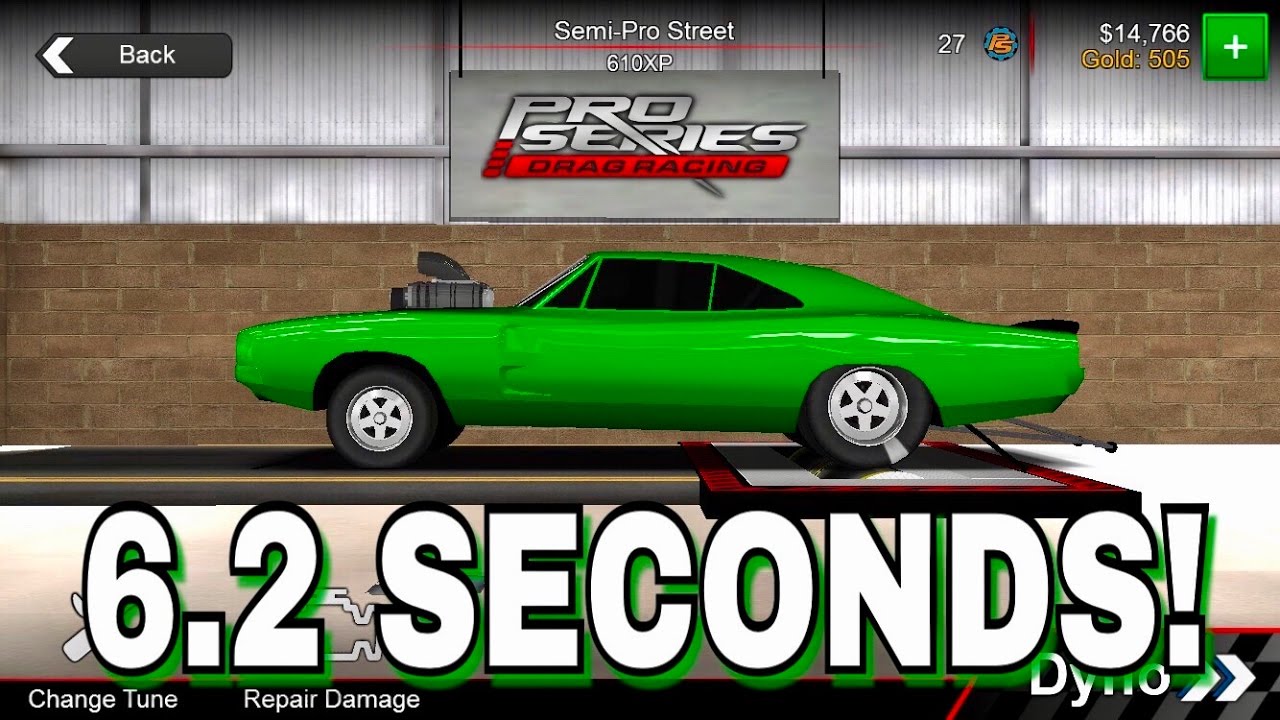The image is a vibrant graphic design from a game scene centered around a green supercar with a massive air intake protruding from its hood, indicative of its high performance. The car sits on a grey trailer embellished with yellow and red lines, occupying the center of the design. Surrounding the car is a detailed backdrop featuring a grey-bricked wall, with a white wall adorned with grey bars above it. 

At the top of the image, bold text reads "Semi-Pro Street 610 XP" in white, followed by "Pro Series" in black on a white background, and "Drag Racing" in black text on a red background, with a grey signboard framing the text. To the right, a gold “PS” symbol encircled by a blue gear icon is displayed beside the numbers "27." Additionally, the top-right corner shows a white money symbol with "14,766" next to it, beneath which "Gold 505" is denoted in gold text, accompanied by a green square with a white plus symbol.

Prominently in the center near the bottom of the image, "6.2 seconds!" is inscribed in white letters outlined in black. The bottom left corner features options "Change Tune" and "Repair Damage" in white text on a black background, while the far right displays a grey and white racing flag area highlighted by a red outline, with “Dyno” and two white arrows.

Overall, the scene encapsulates a detailed, intricate snapshot reflecting the dynamic features of the game, underscored by the car's readiness for high-speed action.